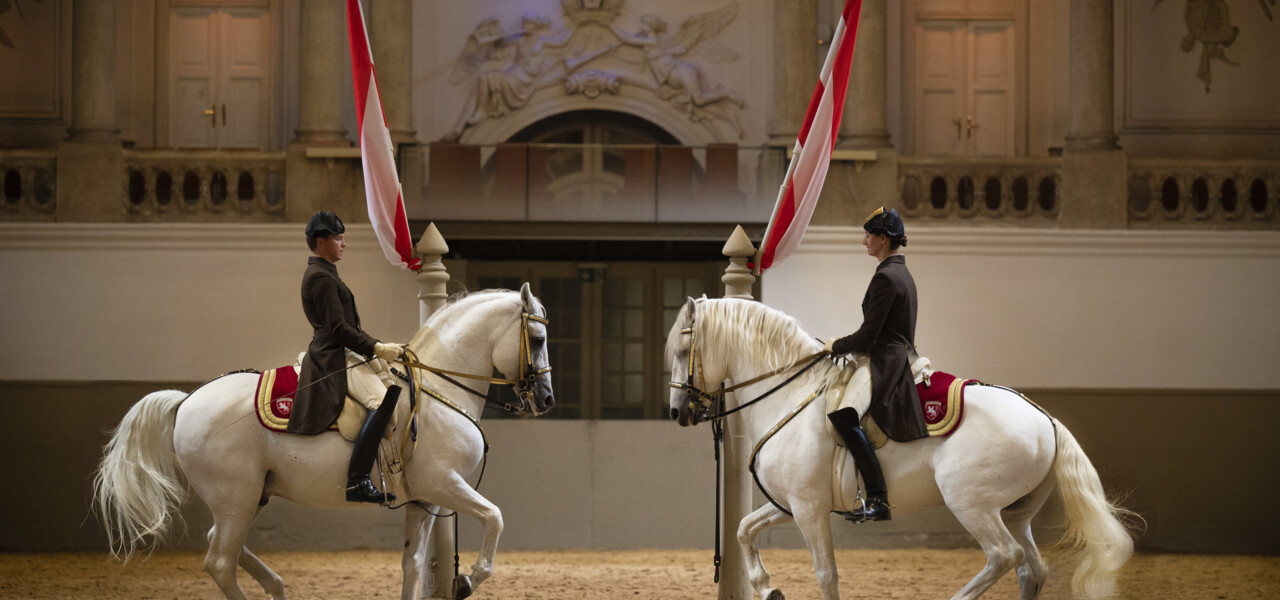This photograph captures an elegant equestrian scene set within a sophisticated, indoor royal arena that resembles the interior of a palace, complete with magnificent columns and ornate white doors adorned with gold handles. The arena's floor contrasts with the luxury, being covered in dirt. Central to the image are two majestic white horses, potentially Lipizzaner stallions, facing each other. Both horses have striking, all-white coats with just a touch of black around their mouths. Adorning these horses are red saddles with gold stripes and logos. The riders, one male and one female, are outfitted in long trench coats that drape down the sides of their steeds. These coats are paired with white riding pants and tall, black boots that extend above their knees. They each wear black caps, and they hold the reins in a relaxed manner. Behind the horses stand two pillars, each displaying a tied-up, red and white flag. The grand backdrop features marble-colored white walls with intricate angel engravings, further accentuating the regal atmosphere.